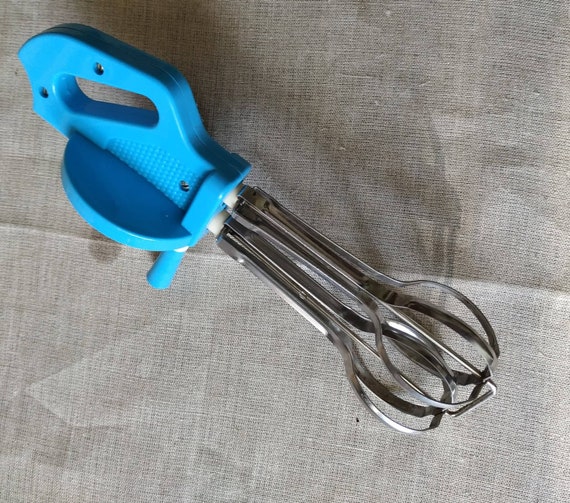This is a color photograph of a manual rotary eggbeater resting diagonally on a crinkled, loosely woven tan linen cloth. The eggbeater features an electric blue plastic handle and crank, secured with three visible screws. The handle is textured for grip, particularly near the hand crank area, enhancing its functionality. The metallic whisks at the base are silver and cast subtle gray shadows onto the cloth beneath. The linen sheet, with its distinct folds and wrinkles, adds a textured backdrop that contrasts with the smooth, shiny surfaces of the eggbeater, enhancing the visual depth of the composition.